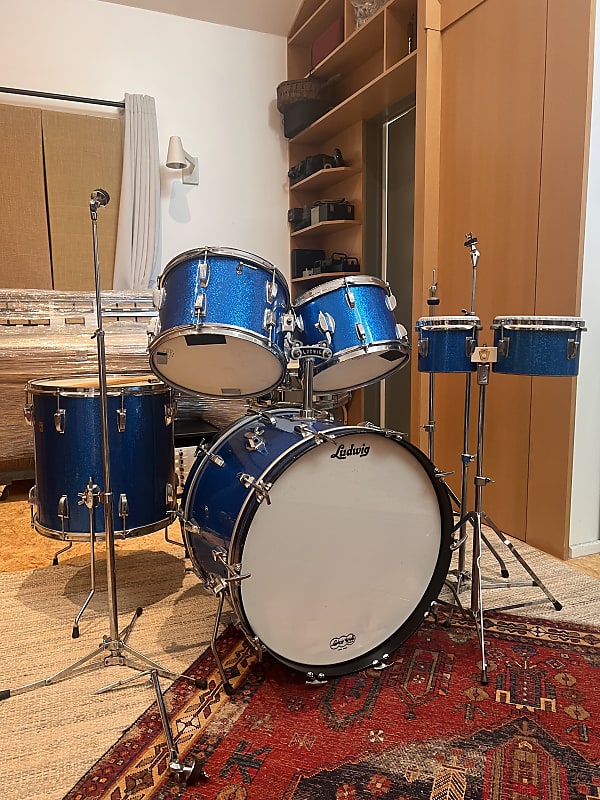This digital photograph captures a complete, metallic blue Ludwig drum set situated indoors on a red patterned carpet layered with a plain tan rug. The drum set, which includes a large bass drum and five smaller drums of varying sizes, sits against a backdrop of shelves, a dark beige closet door on the right, and a white wall to the left. A chrome microphone stand, with a microphone attached, stands near the drum set. Adjacent to the drum set, mounted on the wall, is a lamp with a downward-facing shade and a curtain, adding to the unique setting. The area is illuminated subtly, enhancing the shiny metallic finish of the drums, and the presence of diverse colors—white, blue, red, orange, brown, and green—adds to the room's eclectic aesthetic.